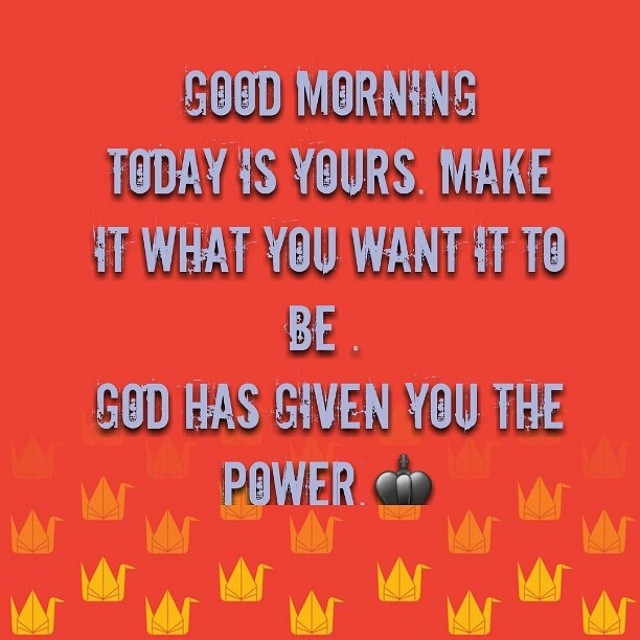The graphic is a motivational poster with a vibrant red background. At the bottom, there are yellow and orange origami cranes, which gradually fade as they ascend. The centerpiece of the image is a grungy, gray font that gives the text an old, roughed-up look. The text reads: "Good morning, today is yours. Make it what you want it to be. God has given you the power." Accompanying the text is a dark gray symbol resembling a pumpkin, or possibly a crown with a cross on top, positioned next to the word "power."